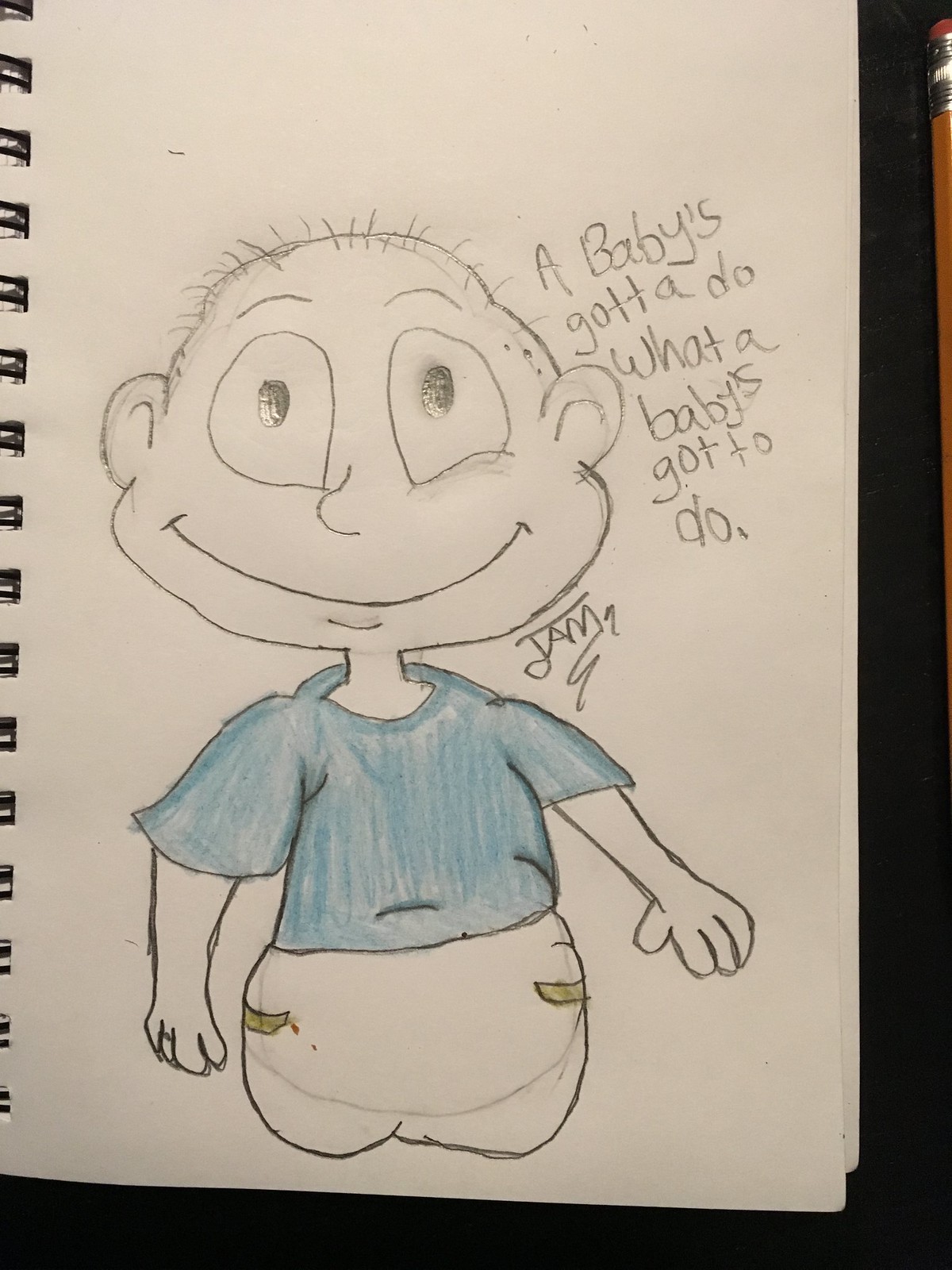A beautifully crafted, creative sketch displayed on a spiral notebook sketch pad. On the left-hand side, intricate spirals enhance the composition. The artwork features a delightful cartoon depiction of a baby’s head, radiating charm and joy with a broad smile, a small chin, and minimal hair on top. The baby's large, curious eyes exude innocence, complemented by cute ears and small features. The baby is dressed in a green short-sleeved crew neck T-shirt and a diaper secured with adhesive strips. Small, endearing hands and arms further add to the cute appeal. Signed with an artistic signature reading either "Jam" or "Tam," accompanied by a playful scribbly line underneath, this sketch stands as an intriguing piece of art. The delicate detailing is highlighted by the natural texture of the paper, bringing to life each element in this captivating drawing.